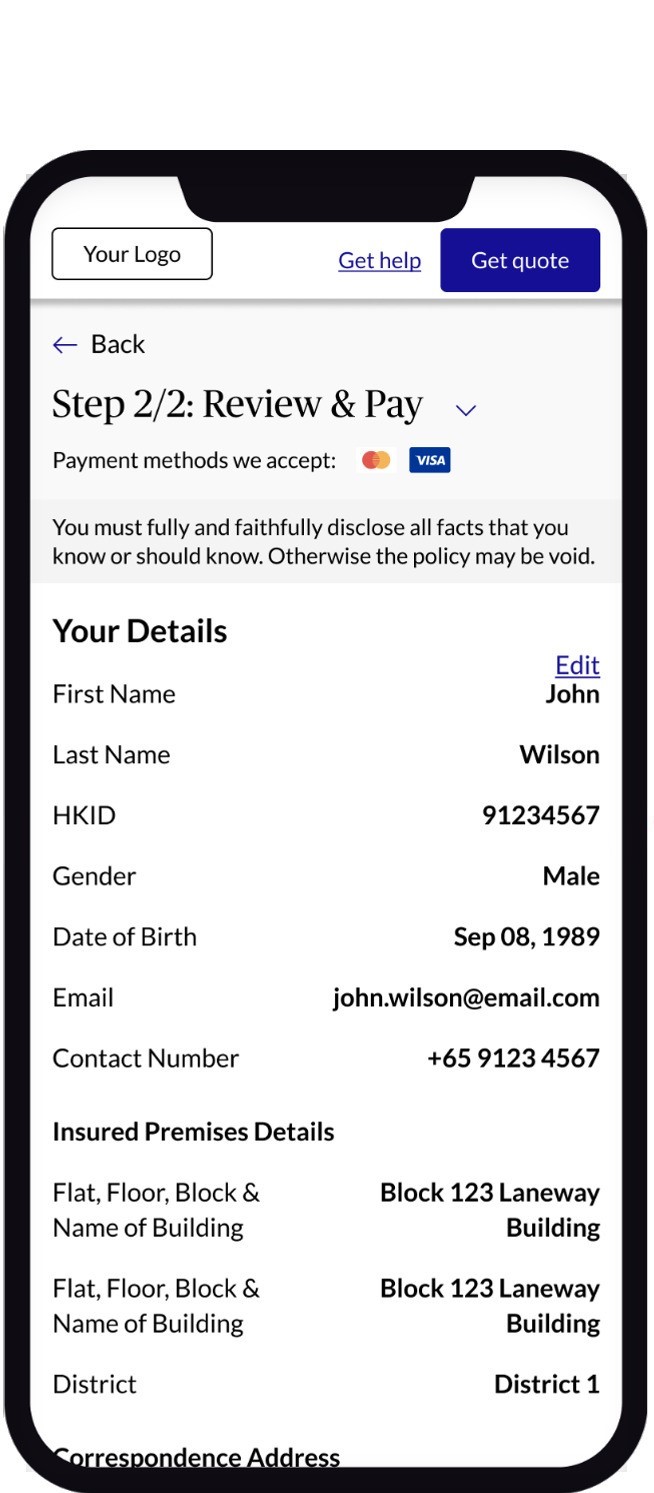An image of a mobile phone screen is depicted with a detailed and functional user interface for an insurance application. 

The phone has a black exterior border, prominently visible towards the top left. Displayed on the screen is a logo with a white background bordered in black on the right side. Below the logo, there is a dark blue, underlined clickable text labeled "Get Help."

Adjacent to this, a rectangular icon with a deep violet background displays "Get Quote" in white text. A light gray shadow serves as a divider, transitioning into a light gray rectangular section at the top left. Here, a left-pointing black arrow is accompanied by the word "Back" in black lettering.

Below this, in a bold black font reminiscent of Times New Roman, the text reads "Step 2-2: Review & Pay." An arrowhead pointing downward indicates an expandable dropdown menu.

The section continues with smaller black text stating "Payment Methods We Accept:" followed by the MasterCard and Visa symbols.

Further down, a medium gray strip contains a cautionary note in black writing: "You must fully and faithfully disclose all facts that you know or should know; otherwise, the policy may be void."

Towards the bottom left, bold black text reads "Your Details," followed by fields labeled in all capital letters: "First Name," "Last Name," "HKID," "Gender," "Date of Birth," "Email," and "Contact Number."

Finally, a bold section titled "Insured Premises Details" contains fields for "Flat/Floor/Block and Name of Building," followed by lines for inputting "District" and "Correspondence Address."